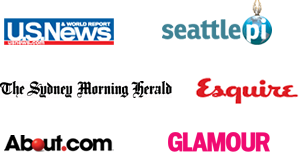The image features six distinct logos arranged against a white background, organized in three rows with two logos per row.

**Top Row:**
- On the left, the "U.S. News" logo is encapsulated within a blue rectangle. The text "U.S. News" is presented in white, with a distinctive red line spanning horizontally across the bottom of the rectangle.
- To the right, the "Seattle PI" logo is set in lowercase letters colored green. Adjacent to the letter "e," there's a green circle containing the lowercase letters "pi" in white.

**Middle Row:**
- On the left, the "Sydney Morning Herald" logo is rendered in bold, fancy black typography.
- To its right, the "Esquire" logo appears in red cursive, featuring a slightly blocky yet elegant font.

**Bottom Row:**
- On the left, the "About.com" logo showcases the words "about" and "com" in bold black type. The letter "O" in "about" stands out as a round red ball, with the dot between "about" and "com" also colored red.
- To the right, the "Glamour" logo is depicted in hot pink, using all-capital block letters.

The overall design is minimalist, focusing attention on the diversity and stylization of each logo.